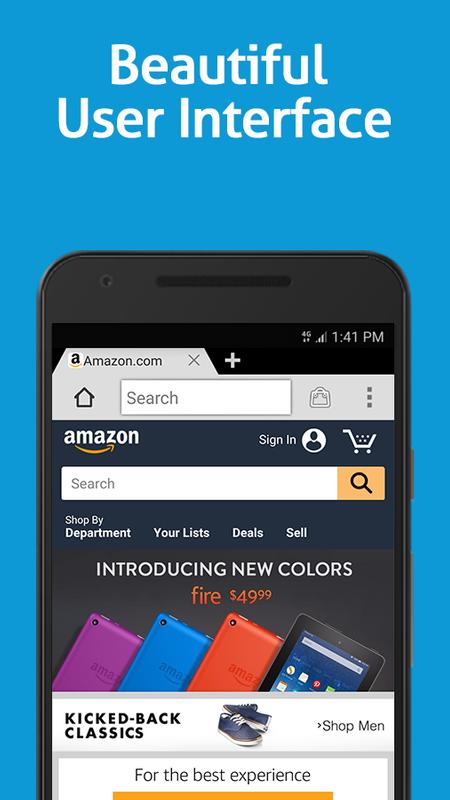The image features a beautifully designed user interface set against a blue background. Dominating the upper part of the interface is a partial view of a smartphone with a black top section. The smartphone screen displays a browser open to the Amazon website, specifically the "Shop by Department" section. The page includes tabs labeled "Your List," "Deals," and "Sell," all in white text against the black browser bar. A shopping cart icon and a "Sign In" prompt are also visible.

The main content of the browser highlights an advertisement for "Introducing New Colors Fire, $49.99." Below this headline, there is a blend of colorful elements showcasing t-shirts, tennis shoes, and other apparel items. The description suggests that the best experience can be gained from shopping for men's clothing. The interface also indicates the current time as "1:41 PM," along with typical smartphone signal bars, 4G connectivity, and a plus sign for adding a new tab. 

The color scheme includes various hues such as blue, white, orange, gray, black, purple, and red, which collectively contribute to the aesthetically pleasing user interface.